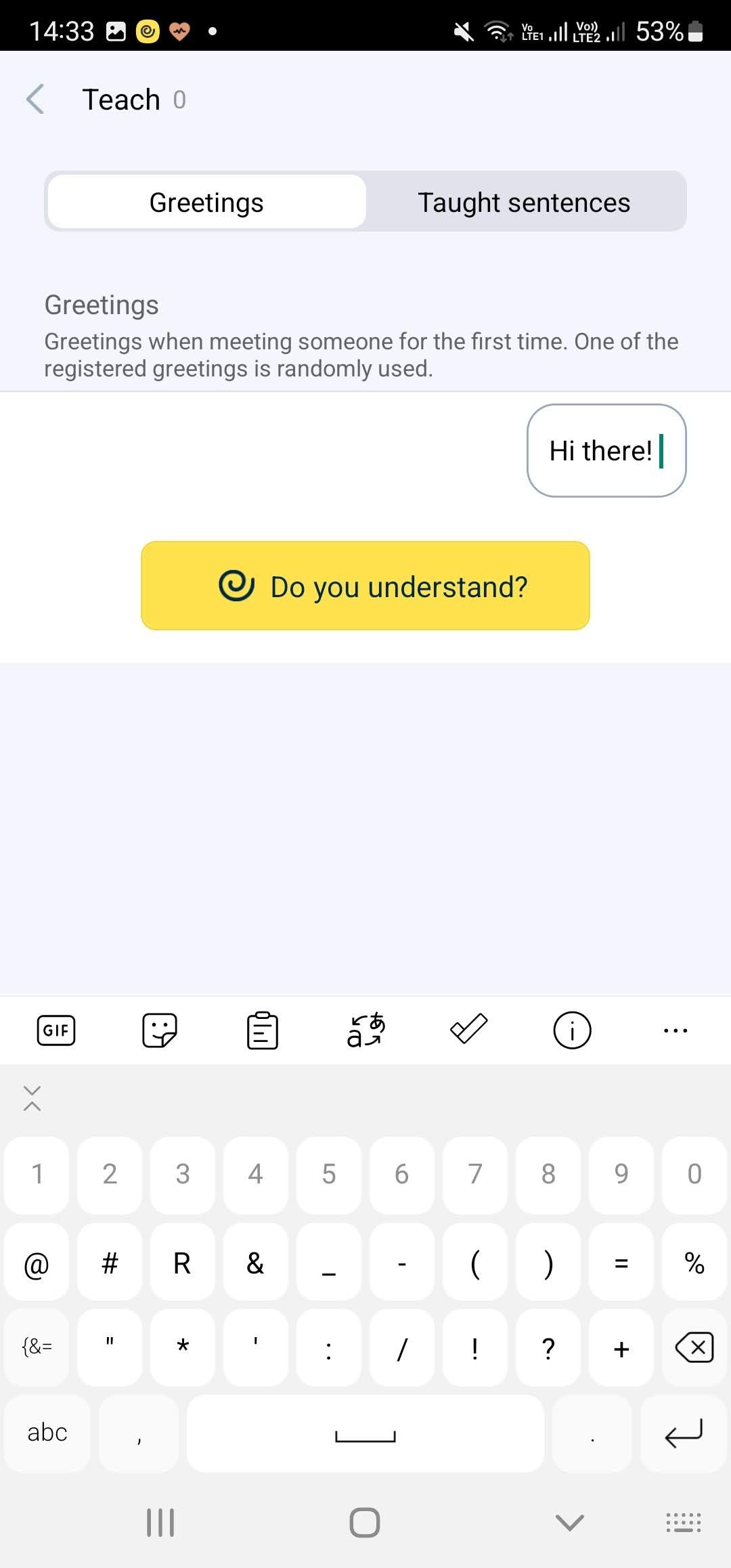The screenshot from the smartphone display captures a detailed interface of what appears to be a language learning or communication application. 

- In the top left corner, the time is displayed as "14:33". 
- On the upper right, the battery is at 53% and the sound is turned off. 
- The header features the word "Teach" followed by a gray numeral zero. 
- Below the header, there are two tabs: a white tab labeled "Greeting" and a gray tab labeled "Taught Sentences".
- The section titled "Greetings" includes a brief description: "Greetings when meeting someone for the first time. One of the registered greetings is randomly used."
- On the left side of this section, a gray rounded rectangle contains the text "Hi there!".
- Following this is a longer yellow rectangle with black text reading "Do you understand?".
- A blank light gray input box is positioned below these elements.
  
At the bottom of the screen are interface icons and a detailed keyboard:
- The top row of the keyboard contains numbers: 1, 2, 3, 4, 5, 6, 7, 8, 9, 0.
- The next row includes special characters: &, #, capital R, &, _, -, (, ), =, %.
- The following row features more symbols: ", *, ,, :, /, !, ?, +, and a backspace button.
- The final row consists of keys labeled "ABC", a comma, a long space bar, a period, and a back arrow.

This comprehensive and structured layout suggests functionality aimed at facilitating text inputs and prompts for interactive communication or learning scenarios.